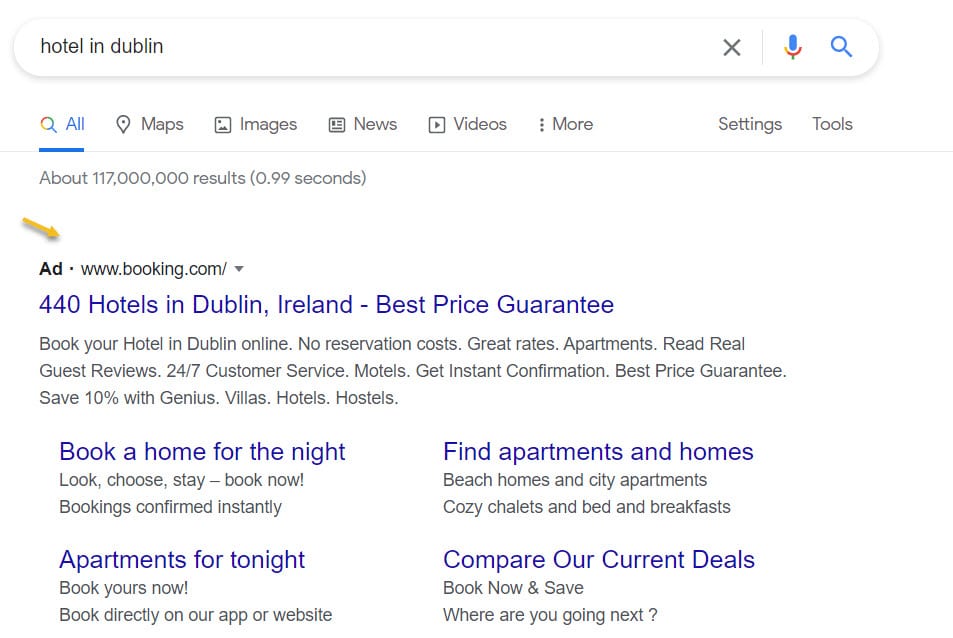The screenshot captures a Google search results page with the query "hotel in Dublin." As is typical, the top of the page displays various navigation options such as All, Maps, Images, News, Videos, More, Settings, and Tools. The search bar, which includes an 'X', a microphone icon, and a search hourglass, indicates the query entered. Approximately 117 million results were generated in 0.99 seconds.

A prominent yellow arrow points to an advertisement from Booking.com, which is the first result. The ad headline reads, "440 hotels in Dublin, Ireland – Best Price Guaranteed," and highlights several features including the ability to book hotels online with no reservation costs and great rates. Additional details mention apartments, real guest reviews, 24/7 customer service, motels, instant confirmation, best price guarantees, saving 10% with Genius, villas, hostels, and options to book a home for the night or find apartments and homes for tonight while comparing current deals.

The image focuses on the Google search layout and prominently highlights the first search result – an advertisement from Booking.com offering comprehensive booking options for hotels in Dublin.